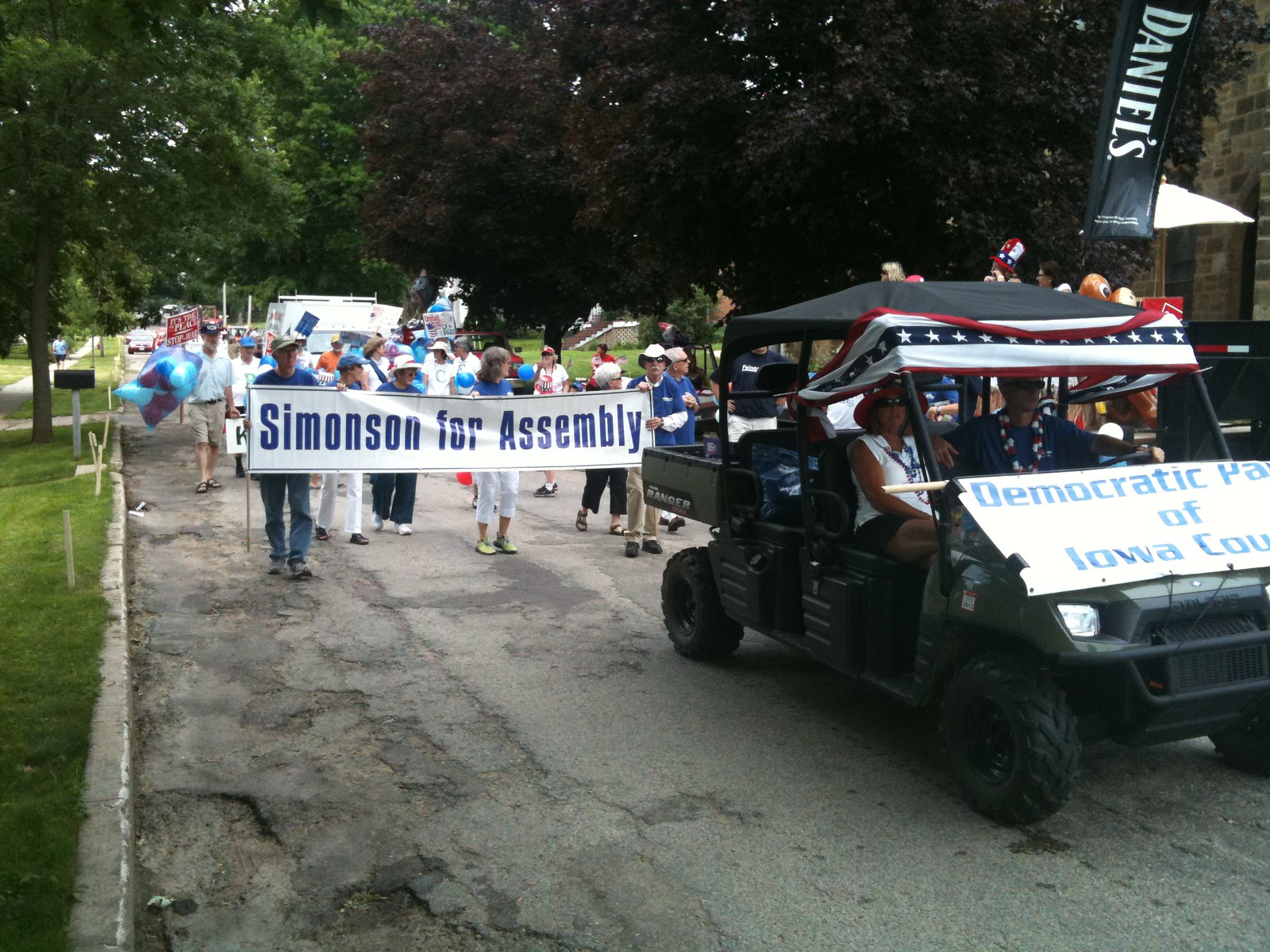The image captures a lively, large square photo of a parade taking place on a worn, narrow street flanked by a neighborhood setting with crumbling asphalt and potholes. On the left side, there's a grassy lawn with a black mailbox on a white pole, indicating a residential area. The street is lined with a mix of green and purple-leaved trees on both sides.

Leading the parade on the right side is a black ATV, resembling a large golf cart with four seats. The ATV bears a banner with American flag colors—red, white, and blue stripes with white stars—and the partially visible text: "Democratic Party of Iowa County." Behind the ATV, there's a large group of parade participants, most of them older individuals. At the forefront of the group are two people holding a prominent white banner with blue letters reading "Simonson for Assembly." 

Among the procession, one man stands out carrying colorful bags of cotton candy, adding a festive touch. Others are holding balloons and additional signs, contributing to the parade's vibrant and energetic atmosphere. The overall scene reflects a spirited community event unfolding in a neighborhood, indicative of both political and social engagement.